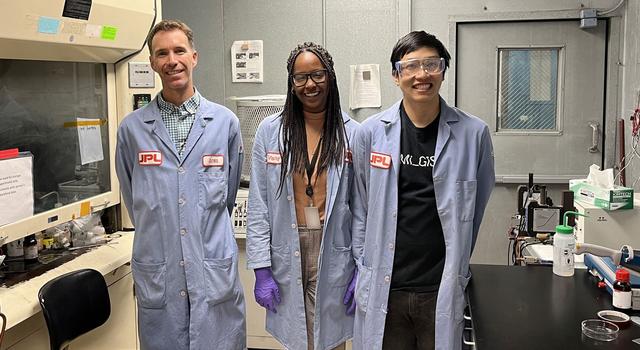This detailed photograph captures a trio of scientists posing in a compact laboratory. Centered in the image, the three individuals are all wearing lab coats adorned with white "JPL" name tags in red lettering. The man on the left, with short brown hair, is draped in a light blue lab coat over a black T-shirt, whereas the woman in the middle, featuring long black hair and dark skin, is equipped with purple latex gloves. She also wears the same JPL coat. The man on the right, possibly of Asian or Hispanic descent, sports short black hair and protective goggles, his blue lab coat worn over a black outfit.

Behind them, the background wall is gray, adorned with some papers. To the far right, there's a door and a lab table cluttered with bottles and tissues. The room’s left corner houses a black chair in front of a cream-colored workstation with sticky notes on the window above it. Other details include a black countertop on the right and the organization of the space, highlighting a functional yet cramped lab environment where these professionals are smilingly posing for the camera.